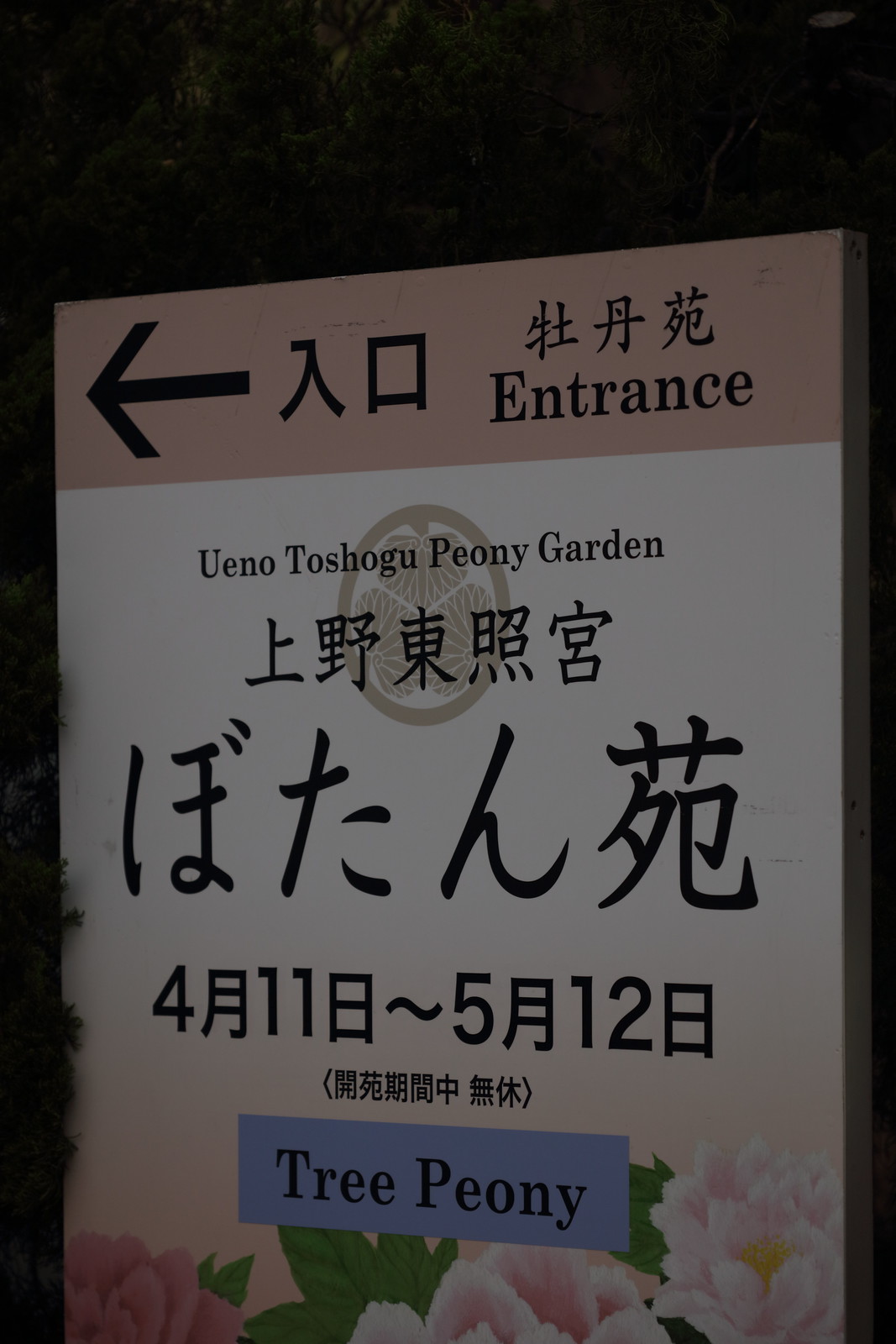The sign is an entrance marker for a garden, primarily written in an Asian language, possibly Chinese. It features a black backdrop and a white main background. At the top of the sign, there is a pinkish stripe with an arrow pointing left, alongside writing that includes the word "entrance" in English. Below, two unreadable words are followed by "Peony Garden" in English. The sign also mentions "Ueno" and potentially "Toshiko." Further down, there are various rows of Asian characters. At the bottom, there are images of pink flowers and green leaves above a blue banner that reads "Tree Peony" in black text. The sign also includes a circular logo with a leaf design.